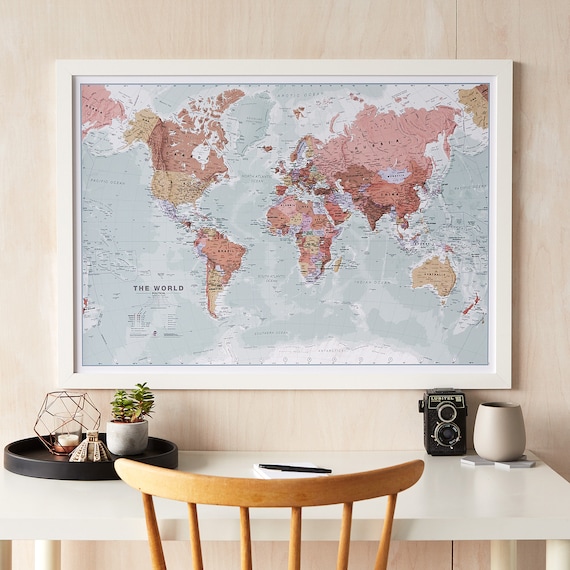This is an image depicting a meticulously furnished room with a focus on a framed map of the world prominently displayed on a light-colored wood wall. The map, enclosed in a thick white frame, showcases detailed continents including North America, South America, Africa, Europe, Asia, and both poles. The landmasses are illustrated in shades of red, tan, purple, brown, and pink, while the oceans retain their traditional blue hue. Above the map, the black letters spell out "The World."

In front of the map hangs a white table with white legs, adorned with a variety of items. A black oval-shaped tray holds a golden wire candle holder with a candle inside, a white pot with a green plant, and other decorative pieces. Nearby sits a piece of paper with a pen on top, and a camera is placed in the right corner. There’s another pot sitting on what appears to be a coaster. Additionally, there’s a mug and a pleasing array of items contributing to the room's aesthetic appeal. A brown chair with visible spindles is placed in front of the desk, enhancing the overall homely and catalog-like ambiance of the setting.